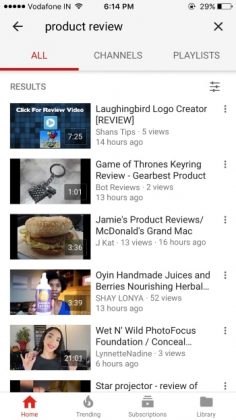This image showcases the mobile version of the Voda app, resembling YouTube's interface. At the top of the screen, "Voda phone" is shown as the carrier, with the current time at 6:14 p.m. Below this, there is a back button situated on the left side and the text "Product Review" centered in the middle. On the top right, a black 'X' icon is available to close the window.

Underneath this top section, there are three tabs: "All," which is highlighted in red and has a red underline indicating it's the currently active tab; "Channels"; and "Playlist." Beneath these tabs, the word "Results" is displayed, along with a filter button on the right side.

Below this header section, there are clickable video thumbnails organized in a vertical list. The videos displayed from top to bottom include:

1. **Laughing Bird Logo Creator Review**
2. **Game of Thrones Key Ring Review**
3. **Jamie's Product Reviews**
4. **McDonald's Grand Mac**
5. **Handmade Juices and Berries Nourishing Herbal**
6. **Wet and Wild Photo Focus Foundation/Concealer**

Each thumbnail provides a snapshot into the available video content, ready for user interaction.